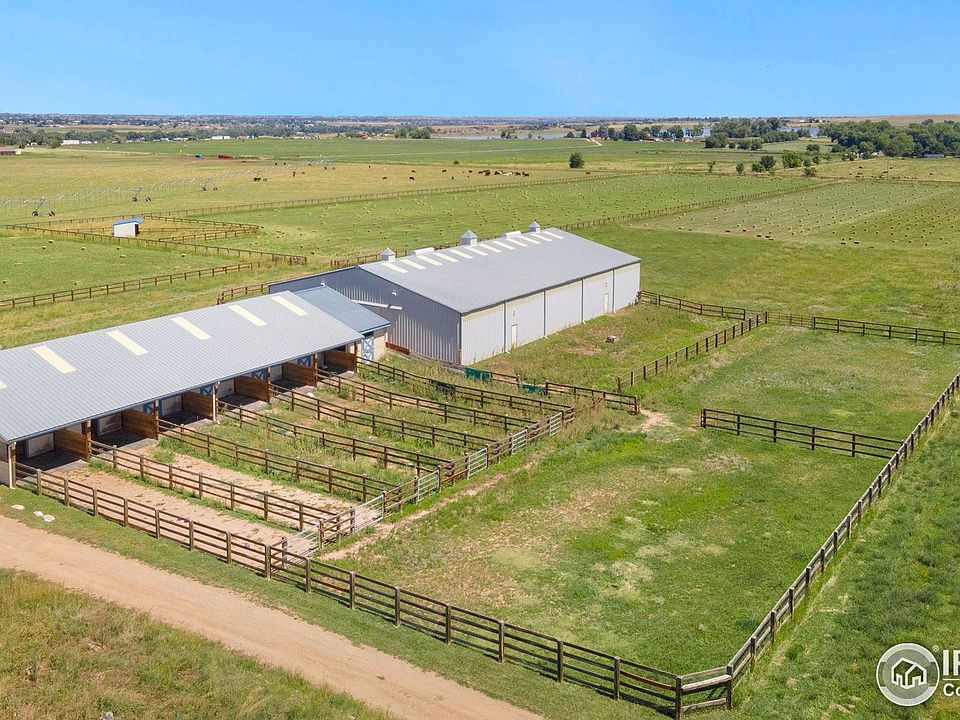In the aerial photograph of the expansive farm, acres of fenced fields stretch out beneath a clear sky. The uniform fencing outlines distinct areas, including two mowed fields where neatly stacked alfalfa bales dot the landscape, ready for storage or sale. Dominating the scene is a large, wide barn, accompanied by a smaller, narrower barn. The smaller barn features multiple stalls, providing spaces for animals to walk out and graze. Adjacent to these structures are three corrals, hinting at the livestock activities inherent to the farm's operation.

Horses populate the scene, with some lying down, others standing, and a few grazing peacefully. Adding to the farm's functionality, an irrigation circle pipe snakes through one of the fields, ensuring the soil remains fertile and productive. Near the edge of the photograph, a small shed with its own corral stands, completing the picture of a well-organized and active farm. The high vantage point, likely captured by a drone, provides a comprehensive view, showcasing the farm's detailed layout and the harmony between its various elements.